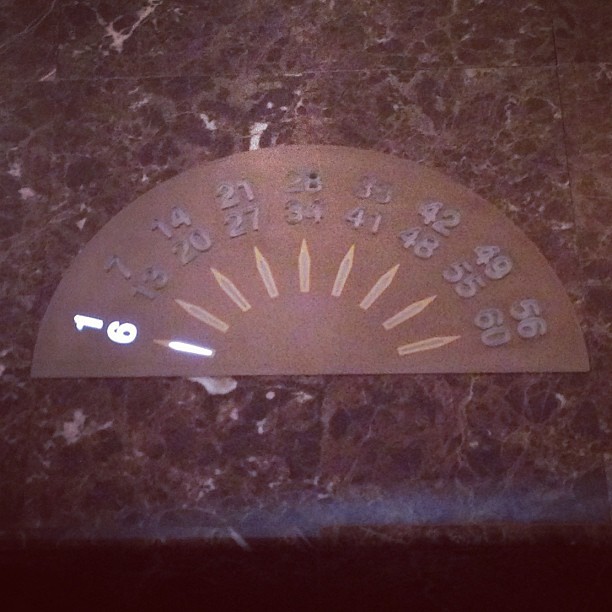A grainy, low-quality, dark photograph captures a section of a wall featuring elevator floor indicators. The image shows a marbled surface with a series of illuminated numbers ranging non-sequentially from 1 to 60. The visible numbers include 1, 6, 7, 13, 14, 20, 21, 27, 28, 34, 35, 41, 42, 48, 49, 55, 56, and 60. Both floors 1 and 6 are currently lit, suggesting the elevator is either on its way down to the ground floor or very close by. The entire scene exudes a sense of anticipation as the photographer presumably waits for the elevator doors to open.